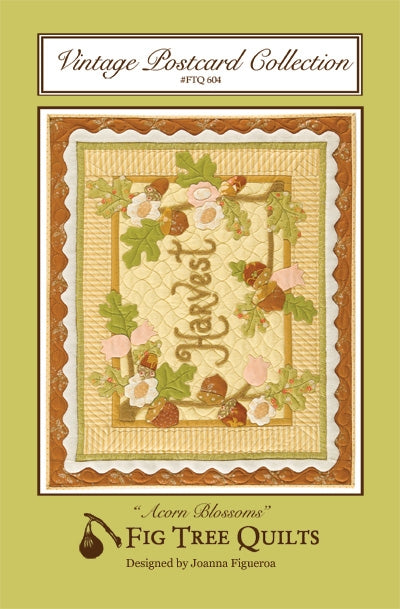This image features the cover design for what is listed as "Vintage Postcard Collection, #FTQ604" at the top in black text on a white rectangle. The primary background color is an olive green. At the center of the image is a slightly tilted photograph of a quilt with a brown border. The quilt showcases the word "Harvest" in brown, surrounded by an intricate design of leaves, pink and white-yellow flowers, and acorns. Toward the bottom of the image, in quotation marks, it reads "Acorn Blossoms," followed by "Fig Tree Quilts, designed by Joanna Figueroa" written in brown. The overall design integrates various elements smoothly, emphasizing the autumnal theme of the quilt and the collection's vintage aesthetic.